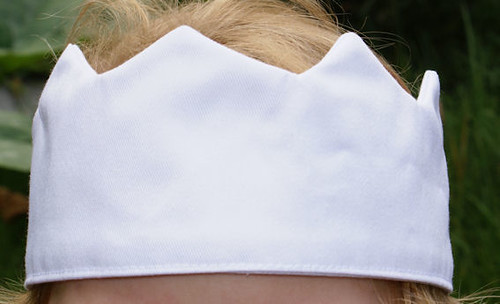This photograph captures the top of a head adorned with a white fabric crown, meticulously detailed with triangular peaks, reminiscent of a playful or makeshift regal headpiece. The individual’s blonde hair peeks out from underneath the crown, with strands pointing upwards and slightly combed back. Visible just below the crown, a small portion of the person's forehead is discernible. The background is a lush green, composed of leaves and grass, contributing to a verdant, natural setting. The image is unsigned, undated, and contains no other elements or people, focusing the viewer’s attention solely on the crowned head and the serene, leafy backdrop.